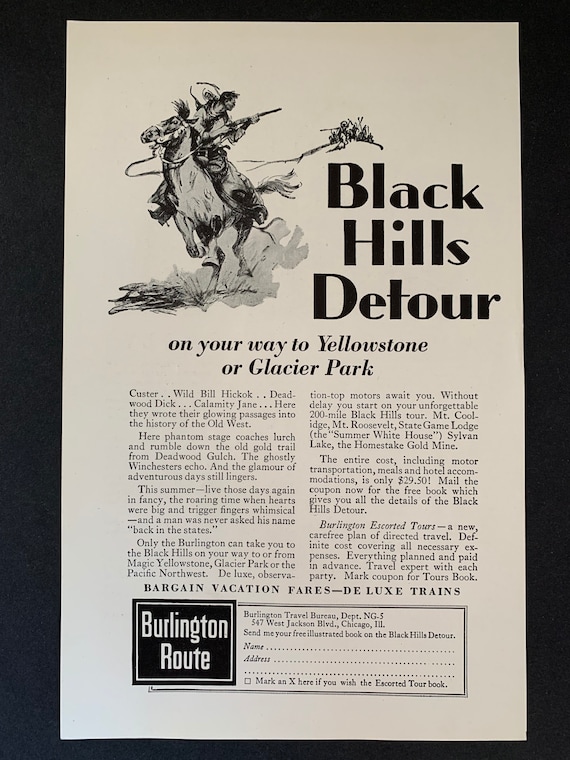The image depicts a black-and-white vintage print advertisement promoting detours through the Black Hills on the way to Yellowstone or Glacier Park. The composition includes an old-fashioned sans-serif title, "Black Hills Detour," printed prominently in black text on a white background. To the left, there is a classic illustration of a cowboy on a galloping horse, wielding a rifle, with smoke and dirt billowing from the horse's feet. Behind him, other figures armed with weapons appear to be engaged in battle, emphasizing the rugged history of the Old West.

The accompanying text nostalgically invites readers to relive the adventurous days of historic figures such as Wild Bill Hickok, Deadwood Dick, and Calamity Jane, where phantom stagecoaches and ghostly echoes of Winchesters fill the imagination. The text emphasizes the romanticized idea of a time "when hearts were big and trigger fingers whimsical and a man was never asked his name."

This advertisement includes practical travel information, including mentions of "vacation fares" and "deluxe trains" via the Burlington Route. At the bottom, there is a section with a black rectangle featuring white text that reads "Burlington Route," beside a form for readers to fill out with their name and address to request more travel information from the Burlington Travel Bureau located in Chicago, Illinois. The entire piece exudes a sense of historical charm and adventure, appealing to those nostalgic for the enigmatic spirit of the Old West.